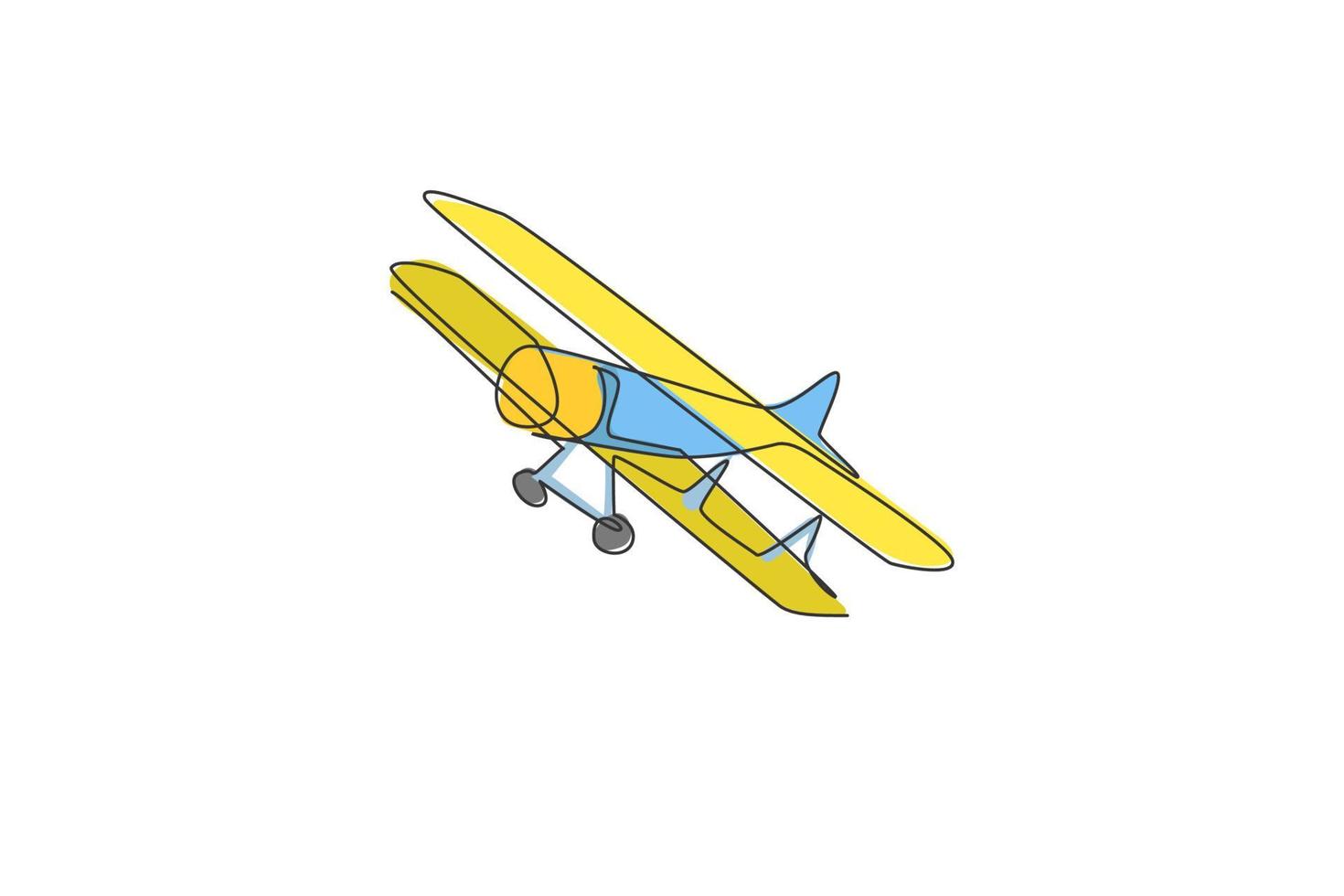The image is a detailed cartoon illustration of a vintage biplane, akin to what the Wright Brothers might have flown. The airplane features two sets of straight wings—one on top and one on the bottom. The upper wings are bright yellow while the lower wings have a greenish-yellow hue. The plane's fuselage is predominantly blue, with the same blue coloring extending to its tail and the metal areas around the structure. Near the front, the airplane transitions into a yellow nose. The barrel-shaped front section is a distinct orange, adding vibrant color contrast to the image. The landing gear consists of small gray wheels, supported by blue and yellow frames that are situated on the angled sides of the plane. Two blue spikes, likely part of the undercarriage, are visible on the bottom wings. The entire illustration is sharply outlined in black against a completely white background, emphasizing the classic design and color scheme of this quaint biplane.